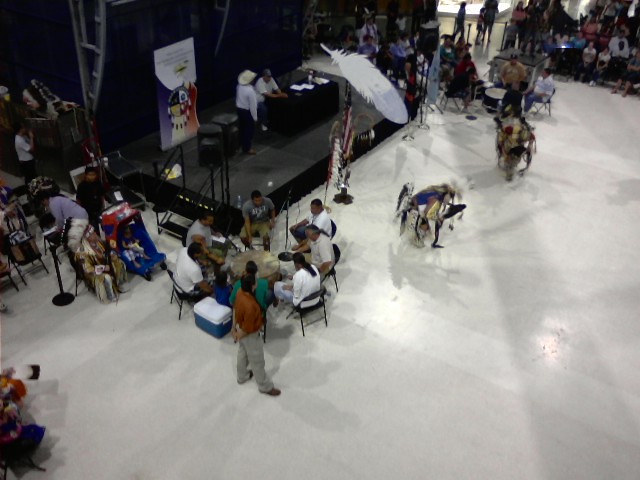The image captures a vibrant gathering of Native Americans or indigenous people within a spacious exhibition hall or auditorium, viewed from a bird's eye perspective. In the top left corner, a black stage is visible, occupied by several individuals seated at a table with fliers behind them. The stage setting appears to be an important focal point, possibly for presentations or announcements. To the right of the stage, a group of Native Americans is seated in a circle around a large tribal drum, dressed in typical modern American clothing, adding a cultural blend to the scene. Adjacent to them, two individuals dressed in elaborate traditional attire are performing a ceremonial dance on a white concrete floor. Further into the background, more people can be seen engaging with drums, enriching the atmosphere with rhythmic beats. A notable figure, potentially a chief, is discernible in one corner, adorned in distinguished regalia. Surrounding the central activities are numerous spectators, encapsulating the communal and immersive nature of the event. Above the scene, a singular white bird feather descends gracefully, adding a touch of ethereal beauty to the bustling, cultural tapestry below.